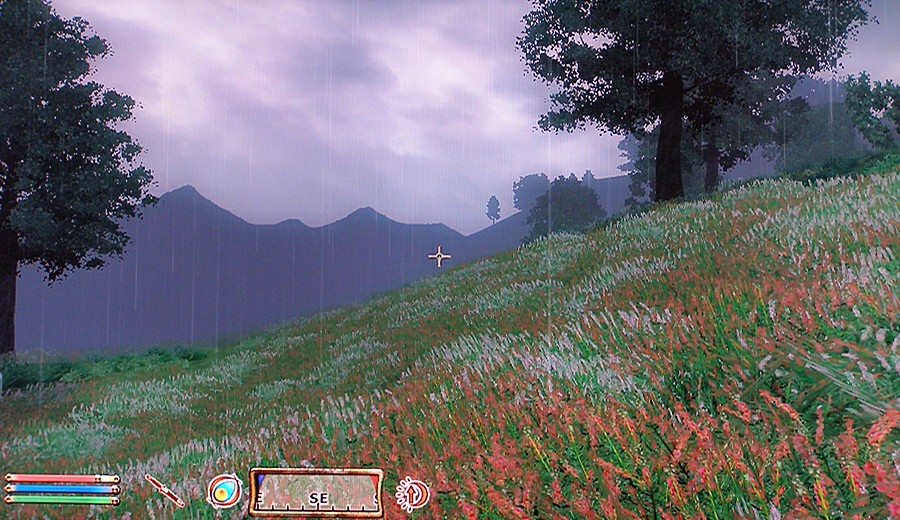This screenshot from a video game presents a detailed first-person view of a grassy hillside terrain. At the center is a white crosshair, indicating the player's focus. The hill features a mix of light green, dark green, and olive green hues, interspersed with red and white splotches that likely represent various flowering plants. On the left side, a dark green tree with a brown trunk stands beside a line of dark green bushes. To the right, more dark green trees and bushes near a mountain display black trunks. The distant silhouette of a mountain is dark gray or black, accented with green at the top.

The scene is set under a gray, overcast sky with visible rain lines, enhancing the moody atmosphere. The lower left corner contains a legend with blue and green rectangles and a partially depleted red rectangle which probably indicates health. Another legend features a red circle within a circle, and an opalescent icon with cyan and yellow. On the right side, a left-facing crescent moon, an upward-facing red arrow, and various multi-colored lines are present. At the center of this display, a rectangle superimposes the player’s area with black hash marks and compass directions ‘E,’ ‘S,’ and ‘SE.’ The grass-covered hillside slants upwards from left to right, with the presence of sparsely placed flowers in purple, pink, salmon, and white colors, adding to the lush, natural setting.